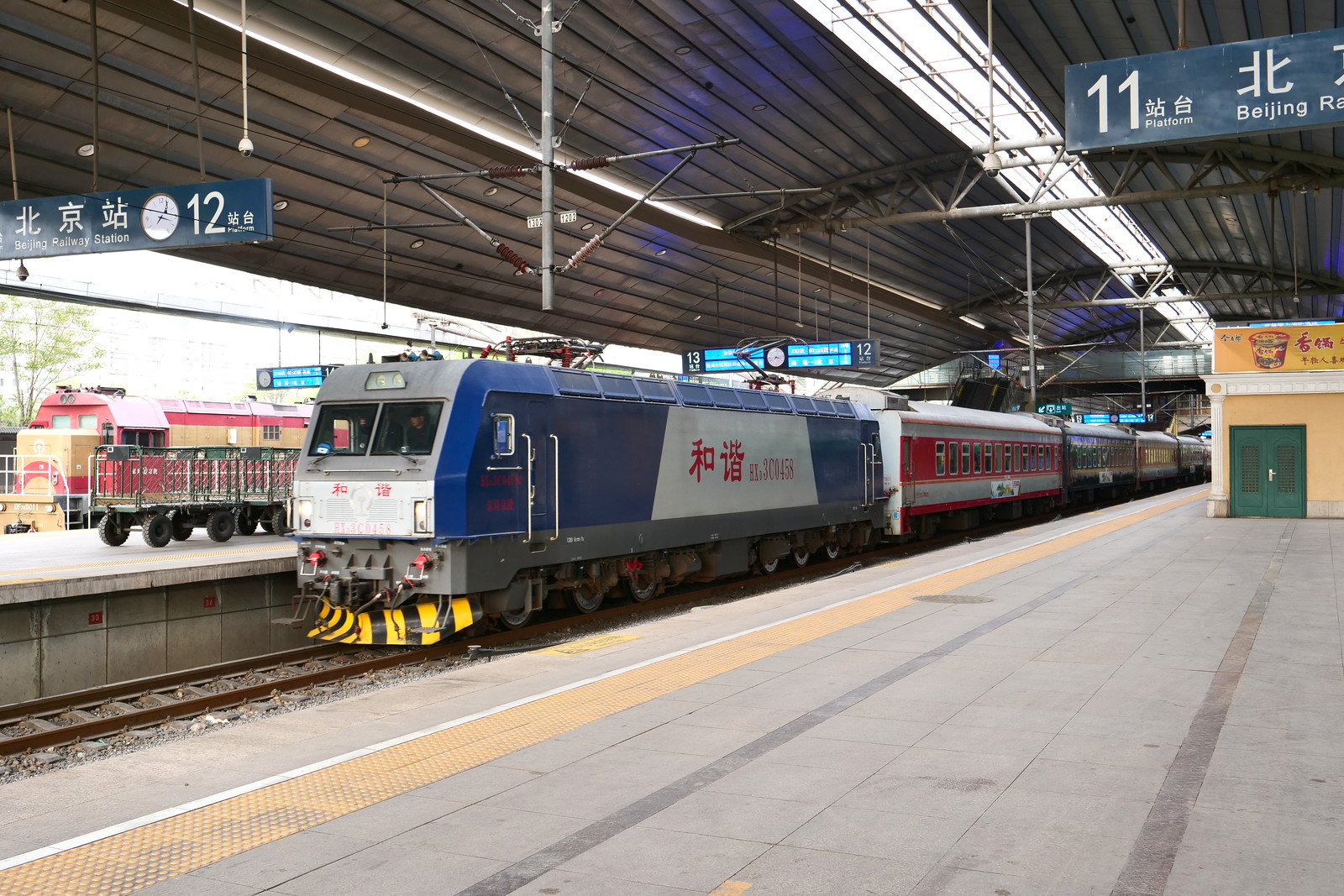The photograph captures a bustling scene at the Beijing Railway Station in China. The station features a curved, gray or silver metal canopy equipped with lights, sheltering the platforms. Prominent blue signs with white writing indicate platform numbers 11 and 12, and accompanying Chinese characters confirm the station name. Dominating the center of the image is a train with a striking black and yellow front, resembling a shovel, operated by a visible driver. The first car of the train is blue and silver with red writing, followed by alternating silver and red cars, and other indistinct cars. To the left, another train with red and yellow features is partially visible. The station's floor is paved with concrete, and a yellow building with green doors is noticeable in the far background, adding depth to the setting. The platform is designed to accommodate passengers boarding the trains, encapsulating the bustling yet orderly nature of one of China’s busy railway hubs.